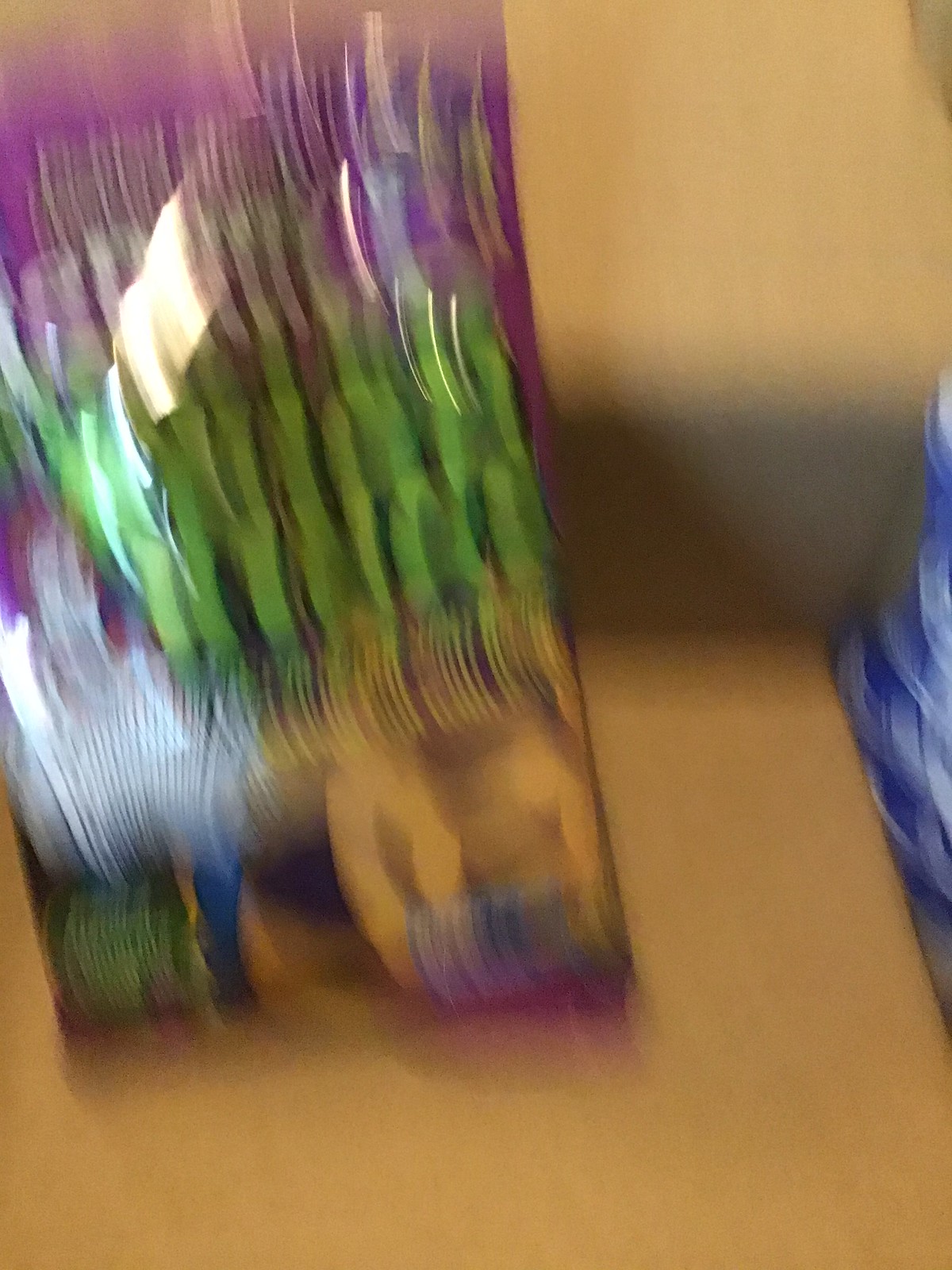This highly blurred image captures a light tan-colored countertop with a matching wall in the background. On the right-hand side, there is a blue, ridged object that appears relatively tall, possibly a vase, though only its edge is visible. Next to this object, there seems to be a tall cellophane bag adorned with green, purple, white, and orange colors. The smudge at the bottom of the bag resembles a carved pumpkin, suggesting it might be a Halloween trick-or-treat bag.